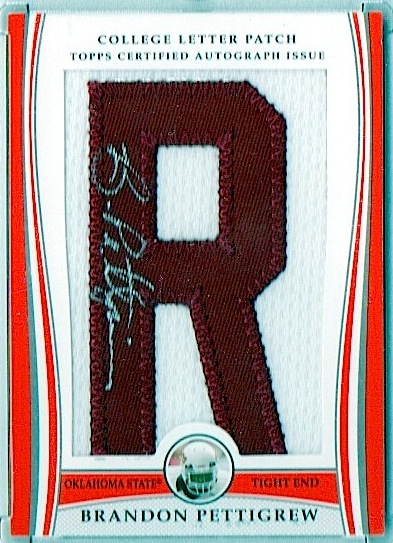The image displays a letter patch for a sports team, specifically for Oklahoma State. Encased in a clear acrylic case, the patch features a meticulously embroidered, maroon R on a white fabric background. The R is personally signed by Brandon Pettigrew, with the autograph, "B Pettigrew," inscribed in cursive.

The top of the image showcases the text, "College Letter Patch, Top Certified Autograph Issue," printed in black or possibly dark blue. At the bottom, “Brandon Pettigrew, Oklahoma State Tight End” is written in black text, flanked by a small picture of Pettigrew himself wearing a football helmet. The name “Oklahoma State” appears to the left of the helmet and “tight end” appears to the right.

Bordering the patch is a vibrant and intricate design comprising red, white, and teal curvy lines that run down the sides, with a combination of red and white lines forming curvy accents at the bottom. The top border is predominantly white. This decorative framing enhances the visual appeal of the letter patch, making it a standout collectible item for any sports enthusiast or memorabilia collector.